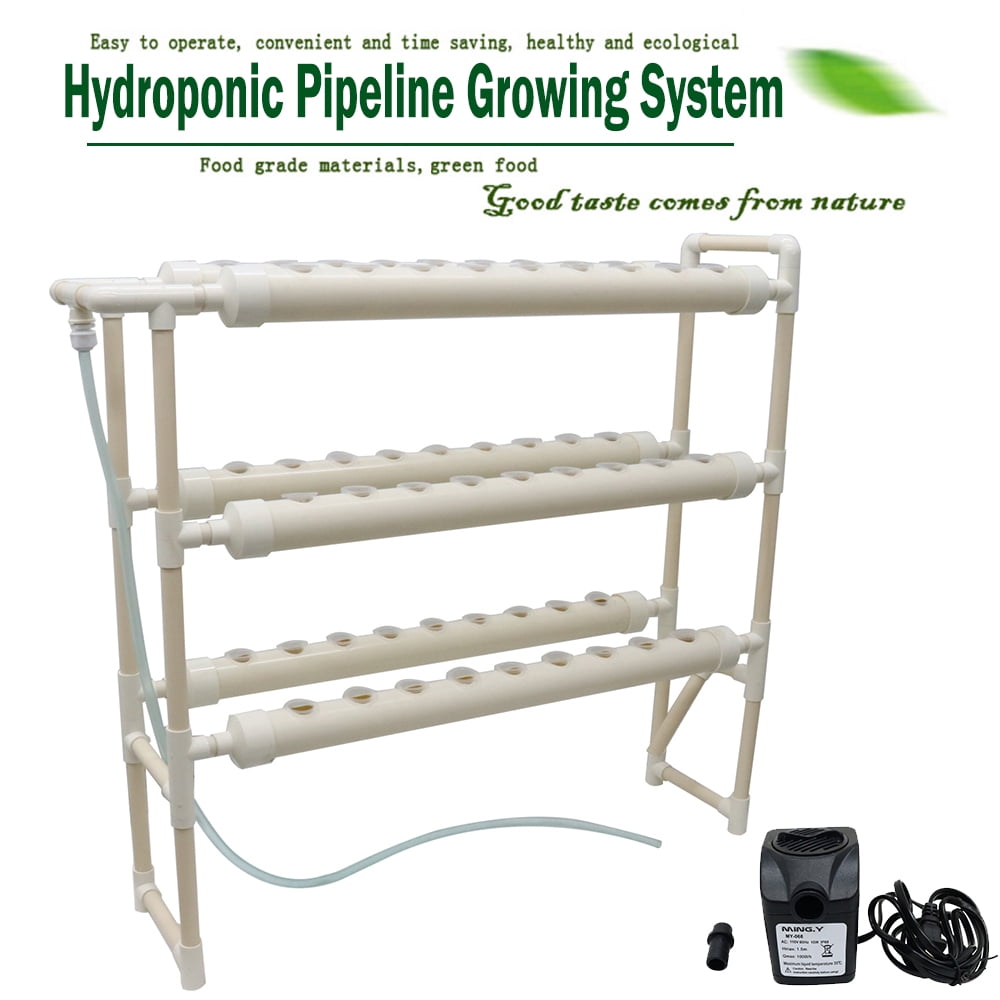The image is an advertisement for a hydroponic pipeline growing system, designed for efficiency and sustainability. At the top, in green text, it reads: "Easy to operate, convenient and time-saving, healthy and ecological." Below, in larger font, it says: "Hydroponic pipeline growing system, food grade materials, green food, good taste comes from nature." The device, primarily made from white PVC pipes, resembles a shelf structure with three levels. Each level features two horizontal cylindrical pipes with evenly spaced holes for planting. At the top of the system, a bluish tube runs down to the bottom. The bottom right corner houses a black rectangular pump with a white label marked "Ming V" and an indecipherable smaller text. Additionally, a long power cord is connected to this pump, indicating the system's capability for circulating water. The background is white, with a slightly blurry green leaf depicted in the top right corner, reinforcing the ecological theme.